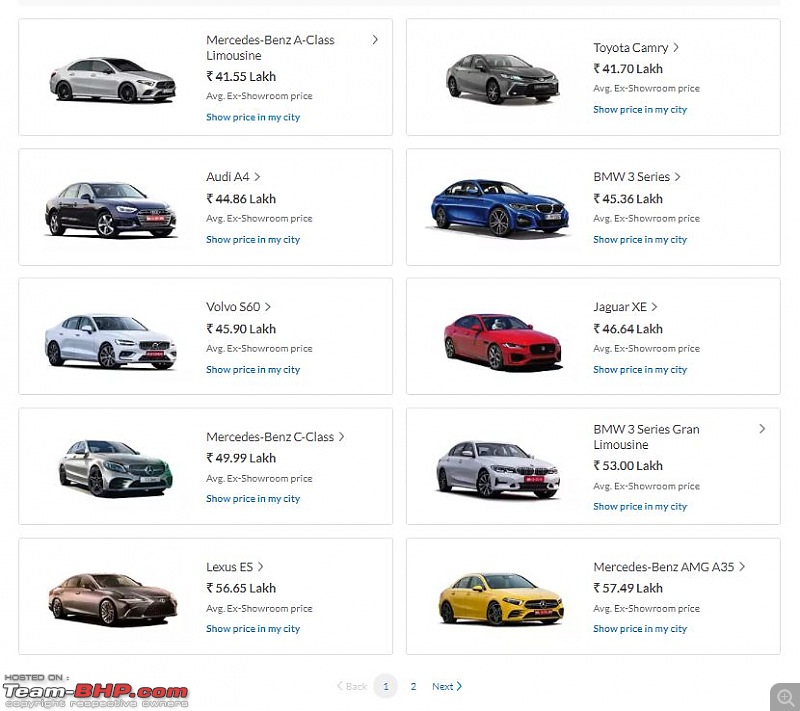The advertisement showcases a variety of vehicles on a website page, split into two columns with five cars each. 

In the left column:
1. **Mercedes-Benz A-Class** at the top.
2. **Audi A4** below it.
3. **Volvo S60** follows.
4. **Mercedes-Benz C-Class** next.
5. **Lexus ES** at the bottom.

Each vehicle is presented with a photo in different colors, and there is an option in blue print labeled "Show price in my city" for each car.

In the right column:
1. **Toyota Camry** at the top.
2. **BMW 3 Series** next.
3. **Jaguar SE** below.
4. **BMW 3 Series Grand Limousine** follows.
5. **Mercedes-Benz AMG A35** at the bottom.

Similarly, each vehicle in this column is also displayed with a photo in various colors, and the "Show price in my city" option in blue is repeated for each.

At the bottom of the ad, there is a mention "hosted on team-bhp.com" from left to right. It also features a navigation bar with a back button, a gray-highlighted number "1" button in blue-green, a number "2," and the word "next" with an arrow, indicating that another page is available for viewing.